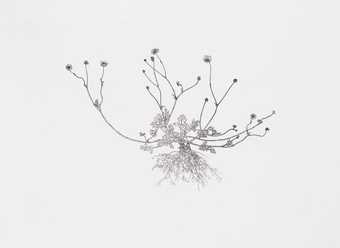The image is a rectangular, width-dominant piece with an off-white, slightly blurred background that resembles a piece of paper. Centrally, there is a detailed black and white, possibly watercolor or ink, drawing that depicts a small herbaceous plant in its entirety. The plant features a main chunky stem from which slender branches radiate outwards in a rounded W-shape. These branches, spread like uplifted hands, are adorned with bead-shaped buds at their tips. The plant, possibly an herbarium specimen, includes root details at the base, with small, insignificant flowers and fruits adding texture to the illustration.